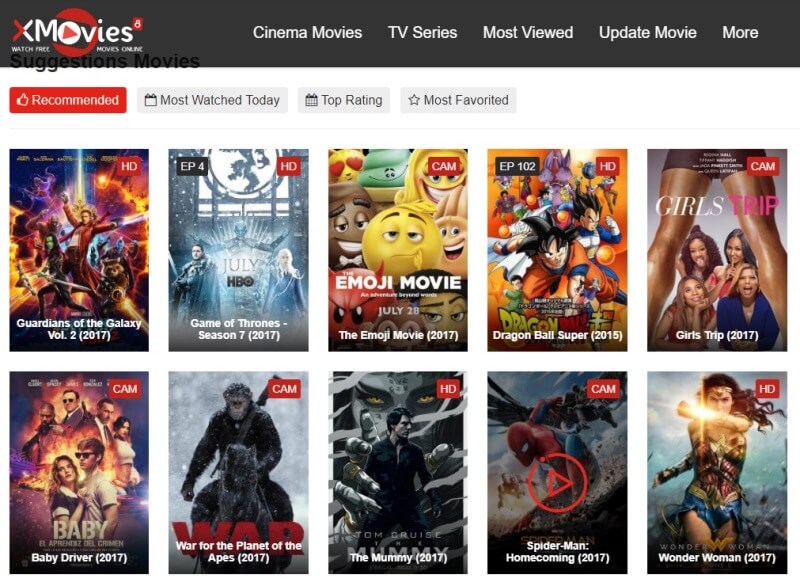At the top of the image, there's a black rectangle containing the text "X Movies." The "X" is split vertically, half red and half white, and the "O" in "Movies" is a circle with an arrow pointing to the right. All other letters are white. There's also a half-circle around the "O" and "B" of "Movies" pointing to the left. Below this header are the words "Cinema Movies TV Series Most Viewed Updated Movies More."

Further down, a row of buttons appears. First is a red button labeled "Recommended." Beside it, there are three gray buttons labeled "Most Watched Today," "Top Rating," and "Most Favored," respectively.

The main body of the image showcases a series of movie posters akin to the covers of DVD cases:

1. **Guardians of the Galaxy Vol. 2 (2017)** - This poster features vibrant, action-packed imagery of the movie.
2. **Game of Thrones Season 7** - A promotional image showing a man with a sword on the left and a woman in a blue gown on the right, with text indicating its HBO release in July.
3. **The Emoji Movie** - Showcasing various colorful and expressive emojis.
4. **Dragon Ball Super (2015)** - Featuring the iconic characters from the Dragon Ball series.
5. **Girls Trip** - Displaying a woman’s legs in black shorts at the top, with four women posed beneath.
6. **Baby Driver** - A striking image with two men in sunglasses in the back and a boy and girl in the front, also with men wearing sunglasses.
7. **War for the Planet of the Apes** - Featuring a solitary ape as the focal point.
8. **The Mummy** - A man flanked by mummies, with white, mummy wrappings streaming across the image.
9. **Spider-Man: Homecoming** - Depicting Spider-Man swinging through the air.
10. **Wonder Woman (2017)** - A powerful image of Wonder Woman in her red, gold, and blue outfit, her hair flowing in the wind, and her iconic tiara gleaming on her forehead.